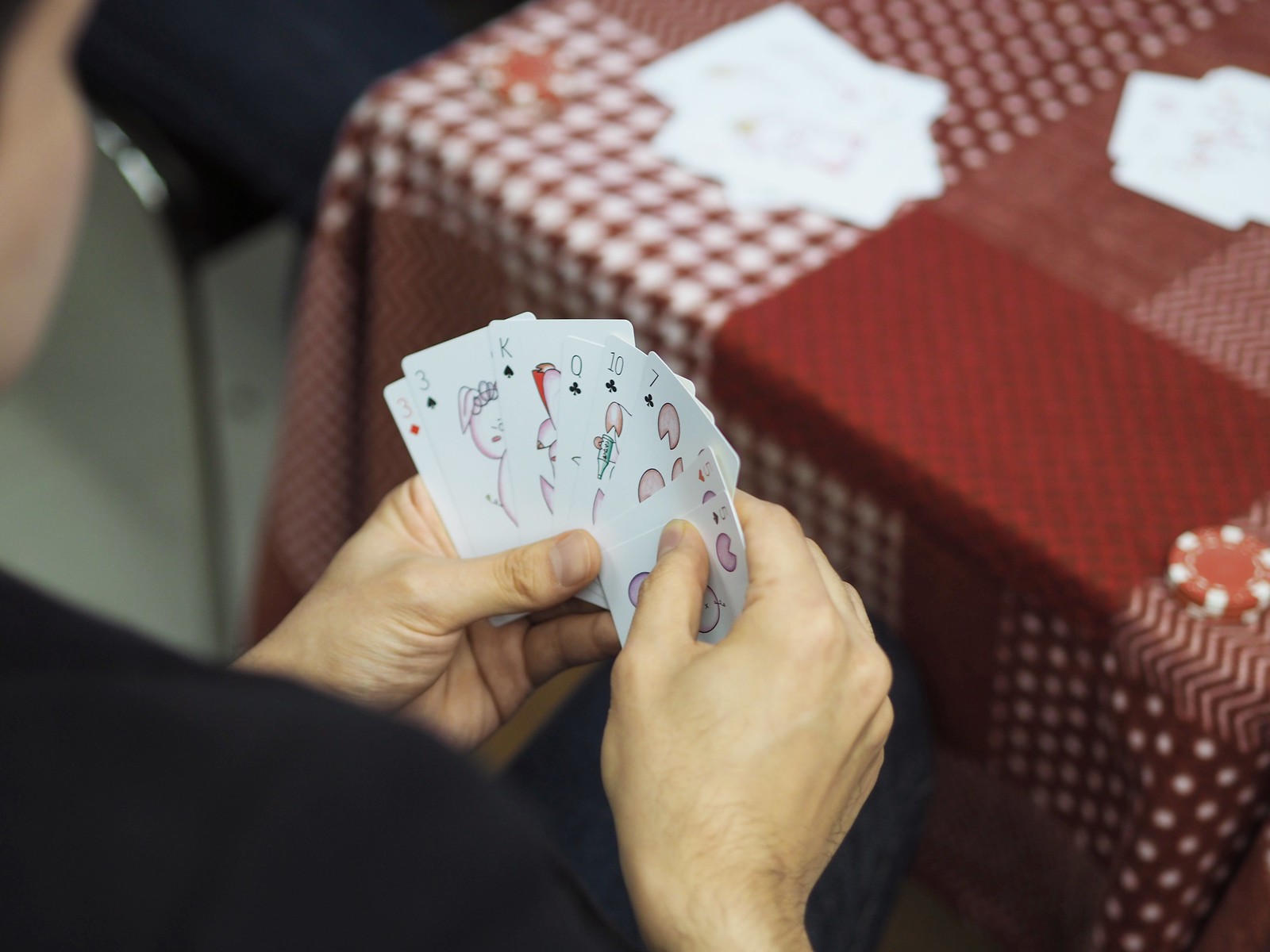A man is intently examining a spread of eight playing cards in his hand, ensuring they are closely guarded from the view of other players. The cards he holds include the three of diamonds, three of clubs, king of clubs, queen of clubs, ten of spades, seven of spades, six of hearts, and five of clubs. The artwork on these cards is unique, featuring distinctive designs rather than the traditional symbols. In the background, part of a playing table is visible, scattered with red poker chips of unknown denomination and a few cards lying face-down. The exact card game being played is not evident, suggesting it could be poker or another variety of card games.